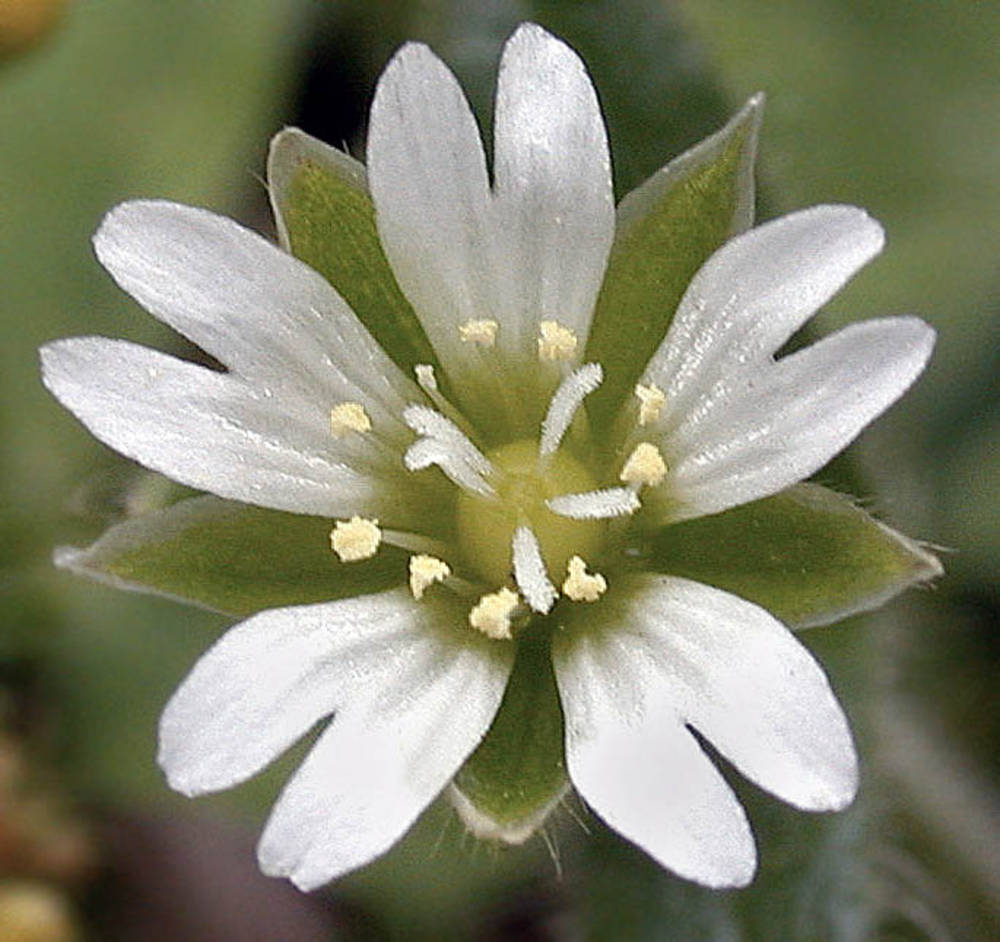This image is a close-up of a striking flower showcasing five pristine white petals, each elongated and heart-shaped with a shiny, delicate texture. Between these petals are five sturdy, diamond-shaped green leaves edged with a soft white border and fine hairs, contributing to a fuzzy appearance. At the center of the flower is a light green core, from which numerous thin, white filaments protrude. Some of these filaments are topped with light yellow pollen, essential for insect pollination. The background of the image is intentionally blurred out, putting the focus entirely on the vivid details of the flower and its features.